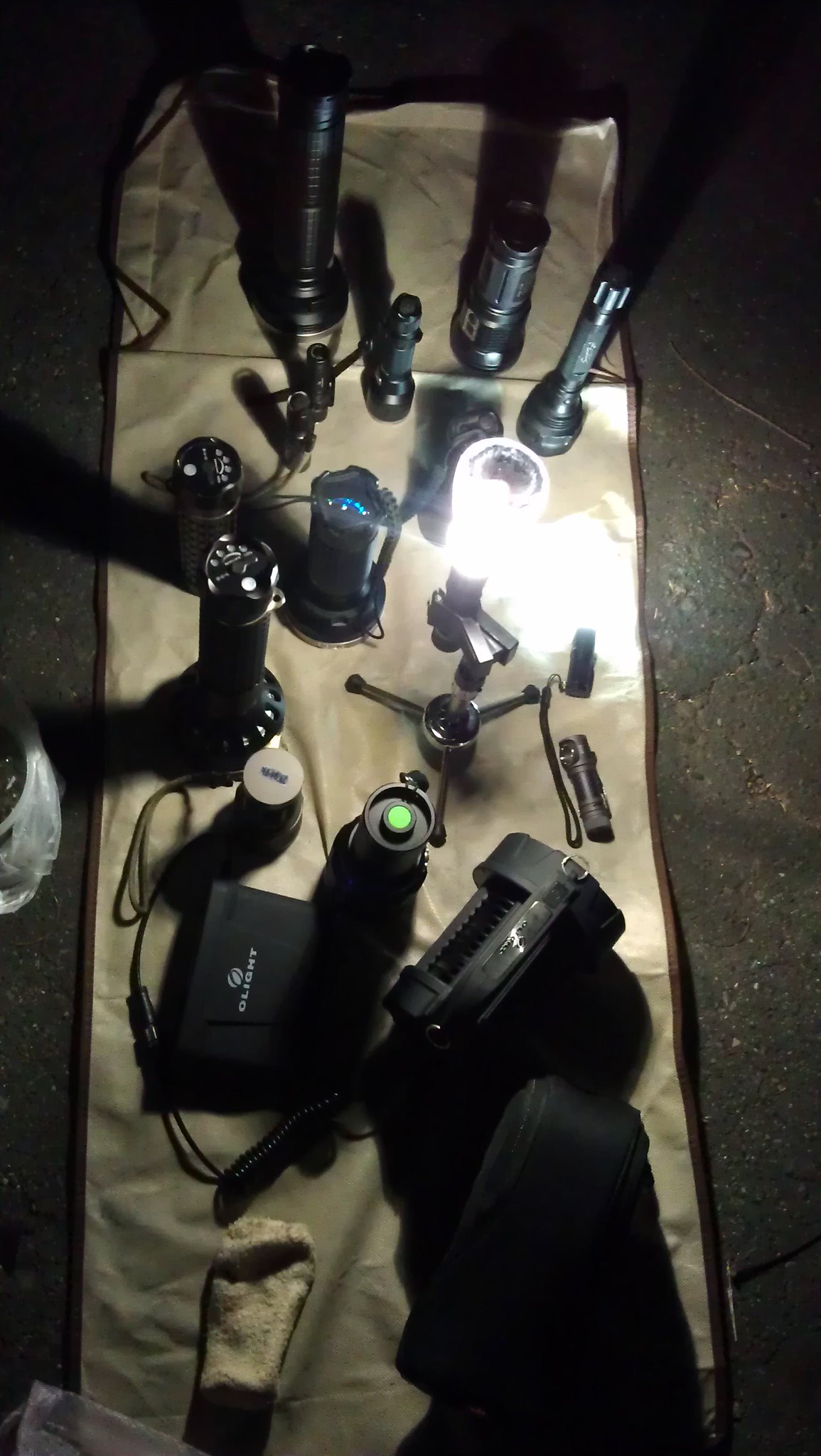This photograph appears to be taken outside at night, possibly in a stony area. The ground is black asphalt, and a long, cream-colored fabric, possibly a towel or sheet, is draped across it. Atop the fabric, there's a variety of black electronic devices, largely consisting of flashlights of different sizes, shapes, and types. Central among these, a lit lantern stands on its base, casting a bright light over the scene. There are multiple cylindrical flashlights, including one big flashlight turned on its side to the right, another upright with a green light, and a smaller flashlight to the left. An additional flashlight on a stand actively emits light, aiding in the illumination of the entire setup. Positioned at the bottom left of the fabric is a rolled-up white or cream-colored object, possibly a cloth or sock. The meticulous arrangement on the fabric suggests a focused, deliberate setup, perhaps for a photography or equipment display, with all elements contributing to an intriguing nocturnal tableau.